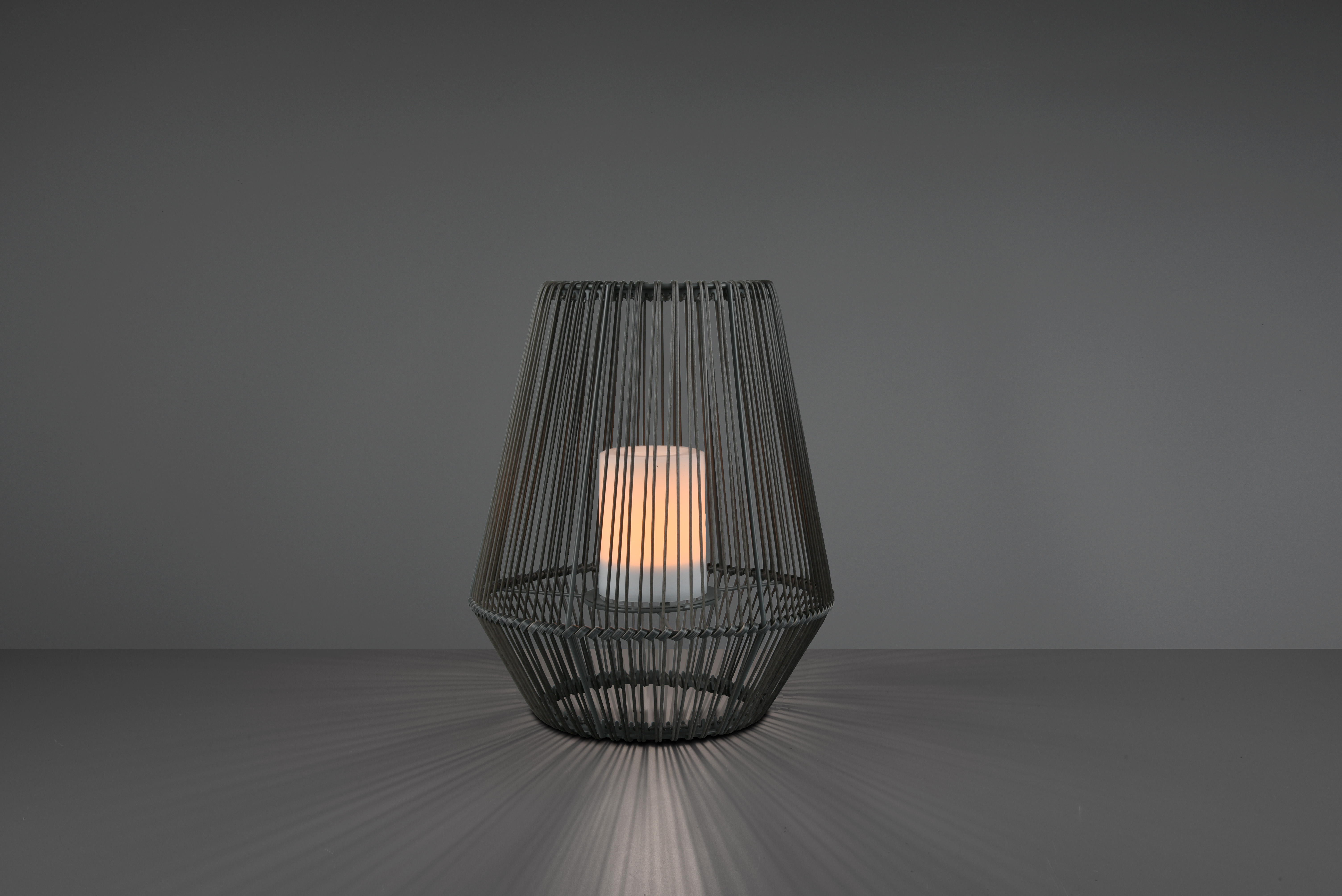In this horizontal rectangular photograph, a sophisticated candle holder is set against a dark gray background with a matching dark gray horizontal surface. The candle holder, crafted from wire, exhibits a unique design resembling a hurricane lamp. Its structure features a bowl-like bottom, reminiscent of a slanted cupcake cup, which narrows towards the middle before expanding into a cone-shaped top that is cut off near the center. This top segment is akin to a slanted lampshade, both parts interconnected by a braided piece of metal. The wire sides, constructed from thick metal threads, allow a lit, battery-operated candle inside to cast a warm glow. This light emanates through the wire mesh, creating intricate shadows on the surfaces around it. The candle sits on a small tray within the holder, illuminating the dark gray surfaces and contributing to the overall elegant and dynamic visual effect of the image.